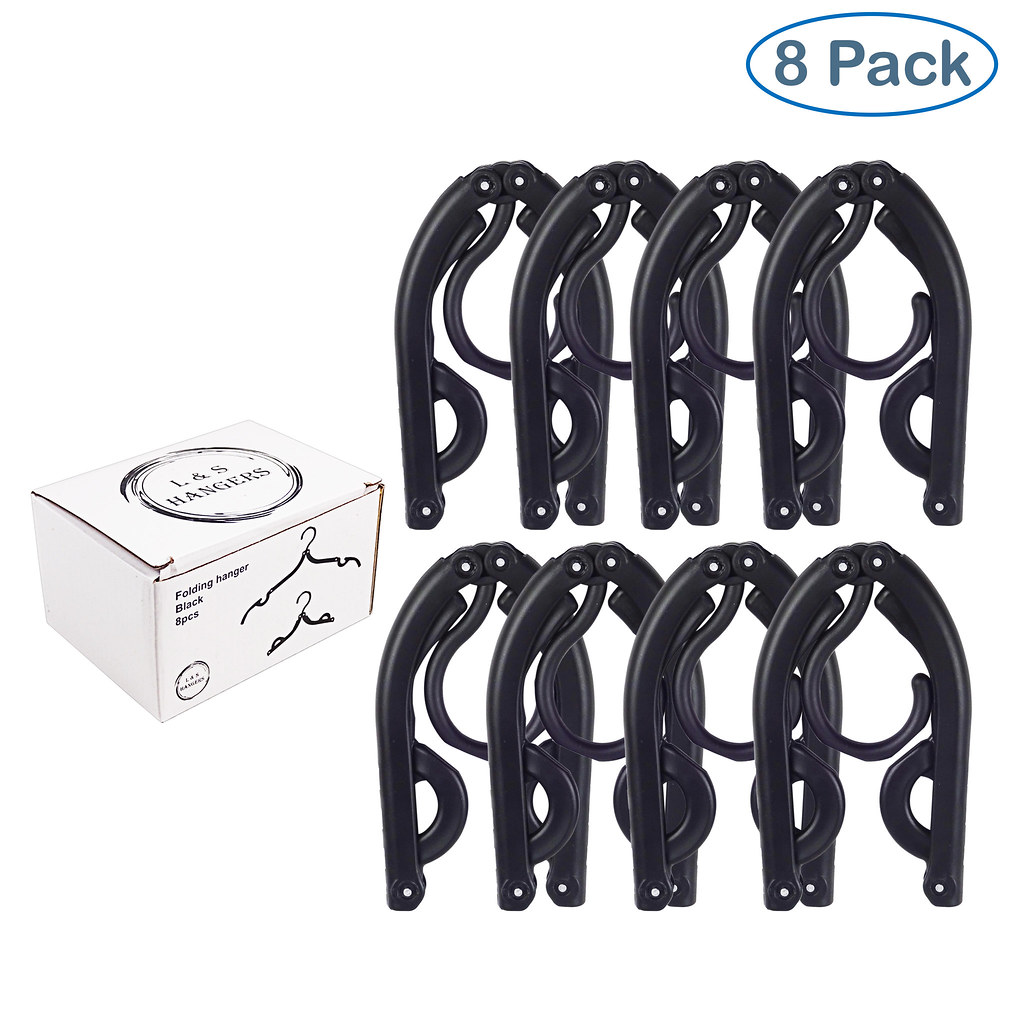The image showcases an Amazon-style product advertisement, set against a white background, featuring a set of black folding hangers. On the left side of the image is a white box prominently labeled "L&S hangers," which depicts the hangers in both their compact and fully extended forms. The box details include "Folding Hanger Black Eight Pieces" and a blue oval label at the top-right corner displaying "8-pack." The foreground presents two rows of four U-shaped black hangers, compactly folded and resembling horseshoes. The hangers are designed to be highly space-efficient, expanding into full-sized cloth hangers when needed. The design includes a plastic curvature within the folded shape, which straightens out to form the functional hanger.